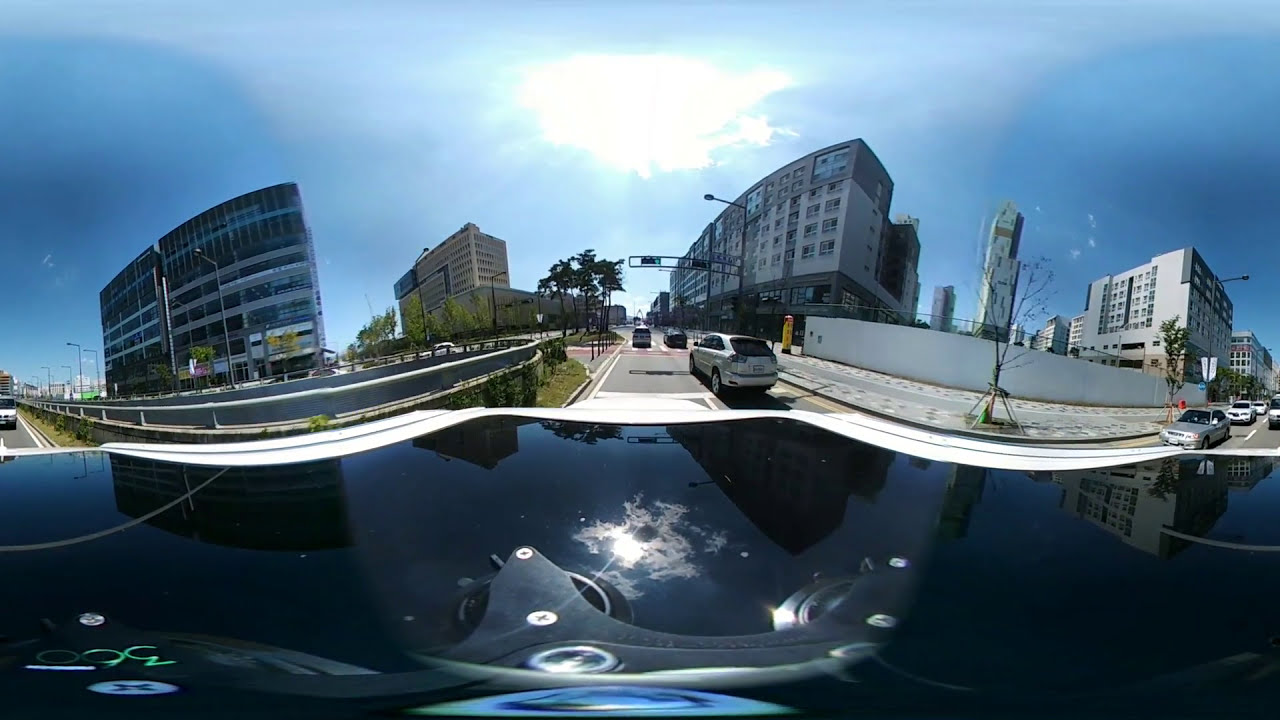The image captures a city street scene viewed from the top of a vehicle's windshield. The scene is framed in a wide horizontal rectangle, with the bottom part of the image dominated by the dark, reflective metal of the vehicle, which gleams under the sunlight. The street ahead is a gray paved road marked by a white center line, with cars driving away from the viewer on both sides.

On either side of the road, there are high-rise buildings, approximately eight to ten stories tall, in various shades of gray concrete. These buildings are interspersed with small trees and patches of grass, hinting at a pleasant, green neighborhood. 

Traffic signals and street lights are visible above the road, which appears slightly curved due to the wide-angle lens used for the photograph, giving the impression of the street bending like the surface of a globe. 

There are three cars directly in front and additional cars to the left and right of the scene. A bridge can be seen further ahead, indicating the end of this section of the road. 

Above the scene is a vast blue sky, mostly clear but for a few hard-to-see clouds, with the bright sun positioned right above the center of the road, casting a strong light over everything.